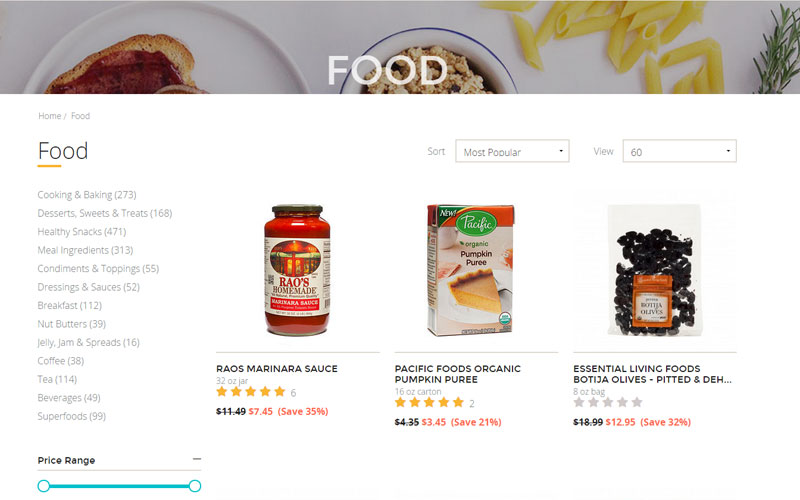In this image, the top header prominently displays the word "Food" against a backdrop that showcases various food items, including a bowl of pasta, what appears to be a bowl of oats, and a plate containing a piece of bread with jelly or jam. To the very left, smaller gray text reads "home/food," and beneath it, the word "Food" is displayed in larger, black text, with a yellow underline beneath the first two letters "F" and "O."

Below these headings is a detailed list of categories and their respective item counts:
- Cooking and Baking: 273
- Desserts, Sweets, and Treats: 168
- Healthy Snacks: 471
- Meal Ingredients: 313
- Condiments and Toppings: 55
- Dressings and Sauces: 52
- Breakfasts: 112
- Nut Butter: 39
- Jelly, Jams, and Spreads: 16
- Coffee: 38
- Tea: 114
- Beverages: 49
- Superfoods: 99

To the right, the image features three food items along with their prices: marinara sauce, pumpkin puree, and boccia olives.